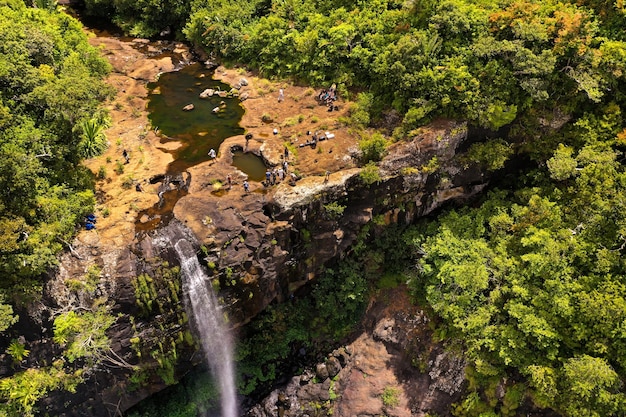The aerial image captures a magnificent waterfall nestled within a canvas of dense, mature green foliage on both sides. The vertically oriented, rectangular frame showcases the tops of numerous trees, spanning from light to dark green hues. The waterfall, starting from the upper left-hand corner, meanders towards the center before cascading down over smooth, dark brown rocks. In the photo, only a modest stream of clear water is flowing over the rocks, hinting at a typically more robust flow. This serene and rugged terrain features a distinct small pool of green-colored water at the top left, edging steeply downwards. Along the very left, you can see the water descending gracefully to the river below. Also visible are many tiny figures of people exploring and walking around the waterfall area, likely drawn by the captivating scenery and the unusually low water flow. This stunning aerial portrayal embodies the essence of nature, intricately balancing the interplay between water and rock.